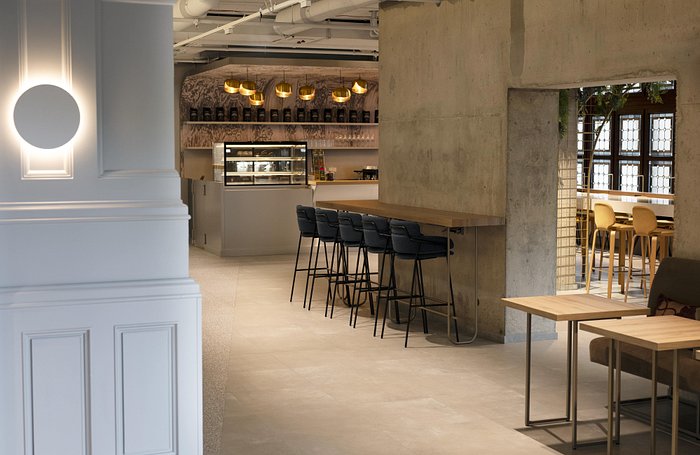The image depicts a spacious and modern interior that appears to be part of a restaurant or possibly a bakery. Dominating the center of the picture is a significant concrete wall with a large stone-like opening that divides the space. Attached to this wall is a counter flanked by five black bar stools, creating an inviting seating area. To the right, another bar stretches across the scene, featuring two lighter brown chairs in the background, adjacent to windows and additional seating.

In the upper middle portion of the image, a counter where orders can presumably be made is visible, though currently unattended, suggesting the establishment may still be under development or not yet open. Behind this counter are two shelves—one holding containers and another displaying what appear to be glasses. There is also a lit glass case on the left-hand side of this counter, which might be used to display baked goods like muffins.

The floor is composed of beige stone or tile, contributing to the natural and earthy aesthetic of the space. Gold lights hang from the ceiling, illuminating the area in a warm glow. Together, these elements create a harmonious blend of functionality and style, hinting at a thoughtfully designed environment that encourages leisurely dining.